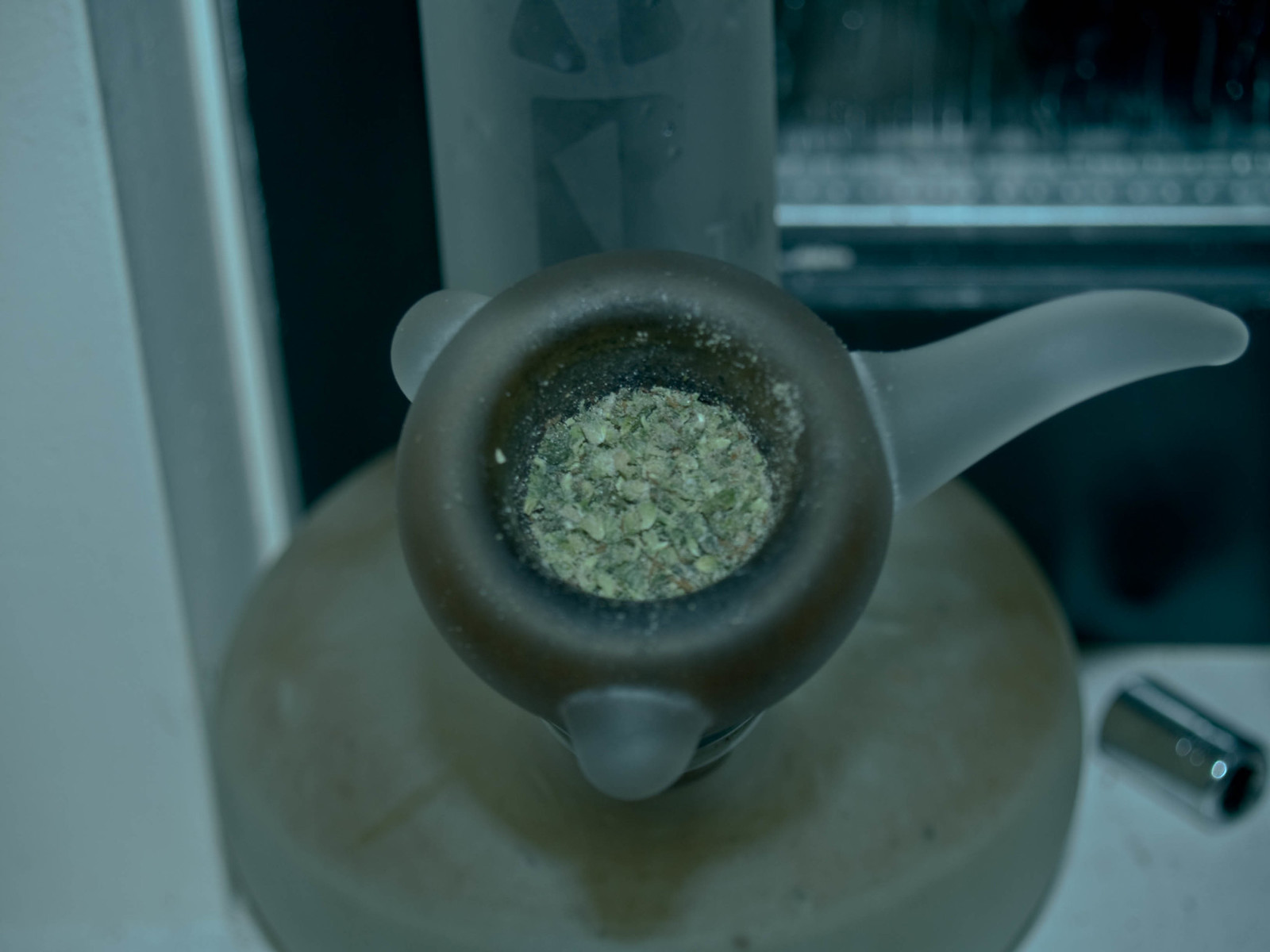This close-up photograph captures a frosted, translucent glass bong designed for smoking marijuana, showcased on a windowsill with a painted wooden border and shiny, stainless steel socket in the bottom right corner. The well-used bong features a matte finish with visible burnt remnants around the edges of the bowl, indicating past use. The bowl, made of frosted glass like the rest of the bong, is tightly packed with finely ground marijuana. The image highlights the three distinctive glass points protruding from the top of the bong, adding to its intricate design, while the background elements such as the sill and metallic socket provide additional context.